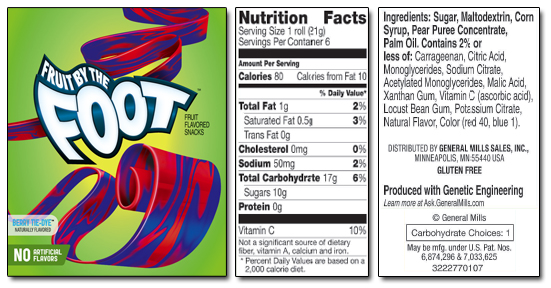The image depicts a computer-generated rendering of the "Fruit by the Foot" fruit-flavored snack, specifically the "Berry Tie-Dye" flavor. The product is presented in three separate images with thin black borders and subtle drop shadows, set against a green background with a bright center and a darker vignette. The central image showcases the product logo, reading "Fruit by the Foot," accompanied by a label that specifies "Berry Tie-Dye" and "No Artificial Flavors." The snack itself is illustrated as a long, ribbon-like strip with a red and blue marbled tie-dye pattern.

The right image features the nutritional facts, indicating a serving size of one roll, with 80 calories per serving, 10 of which are from fat. The detailed nutritional breakdown also includes data on total fat, cholesterol, sodium, carbohydrates, and protein.

The left image displays the ingredients, highlighting the main components like sugar, corn syrup, and fruit puree concentrate, along with various colorings and chemical additives. Additionally, the image provides General Mills Sales Inc. contact information, as well as allergy and GMO disclosures.